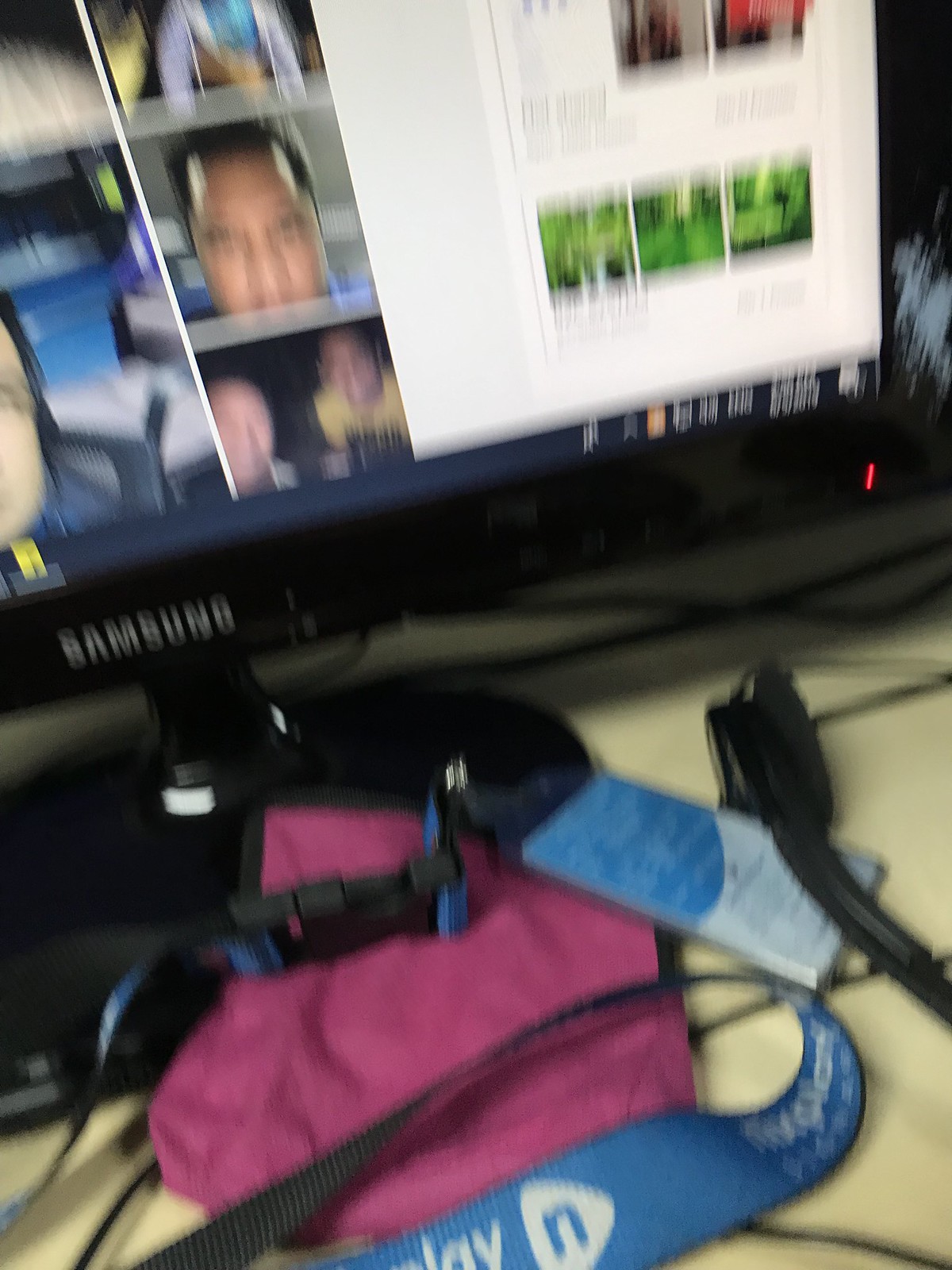A blurred image captures a black Samsung computer monitor displaying various images of people's faces arranged in rectangles, alongside a sizeable white area on the right side of the screen. The monitor, positioned at a slight angle from the left center to the slightly above center on the right side, features a visible red button that indicates it is powered on. To the forefront of the monitor, lying on a light yellow table, is a blue neck holder with white lettering, possibly part of headphones, and a magenta cloth item situated in the lower center portion. The photo is taken vertically in an indoor setting with low light, creating a slightly dim ambiance.